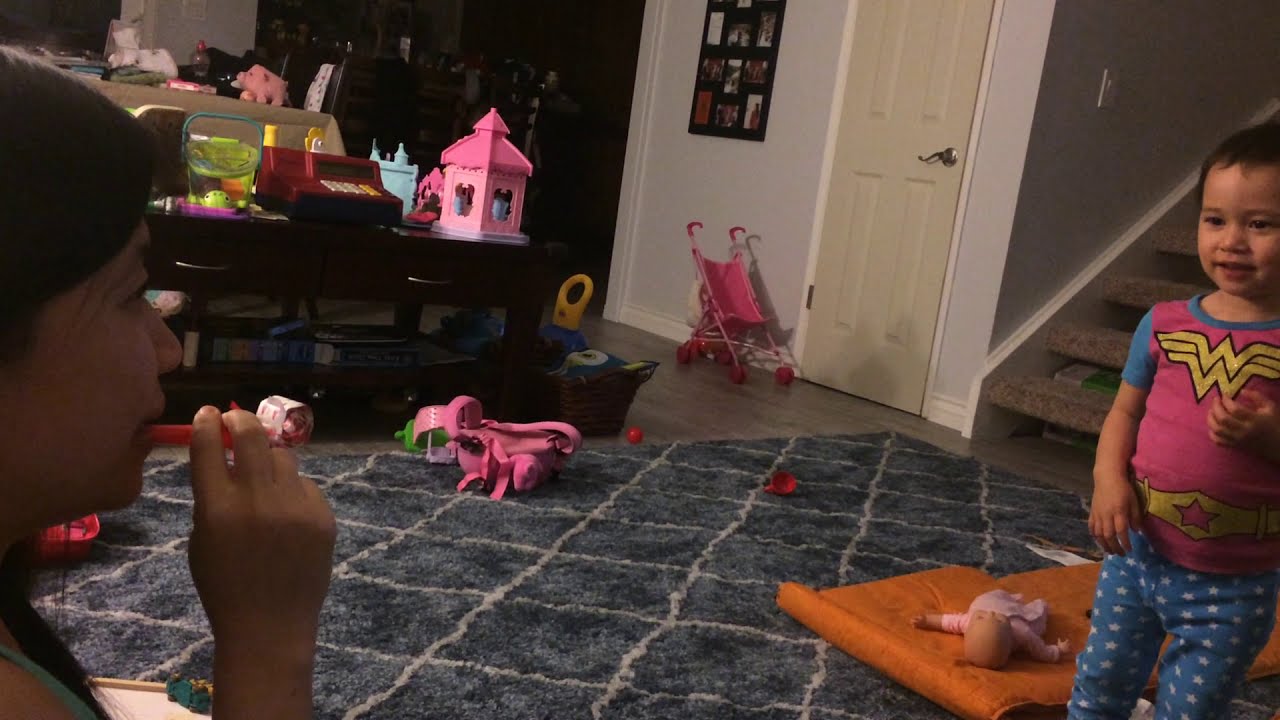The image captures a cozy playroom in a home, filled with various children's toys scattered across a gray and white rug with diagonal stripes. Dominating the scene on the right is a young child around three years old, clad in Wonder Woman pajamas with an emblem and logo on the shirt, paired with blue pants decorated with stars. To the left, an older individual with very dark hair, possibly a parent or caretaker, is caught in a playful moment, poised to blow into a party favor that unfurls when used. This person is facing the child, establishing a connection within the lively scene.

Various elements populate the playroom: a doll perched on an orange pad in the lower right corner, a baby carriage positioned against a white wall near a door with a staircase leading upwards, and a framed collage of photos adorning the distant wall. A table in the back left corner is heaped with toys, including a little pink toy house, while a shelf filled with additional children's toys lines the wall. This snapshot encapsulates a moment of joyful interaction within a warm, cluttered playroom environment.